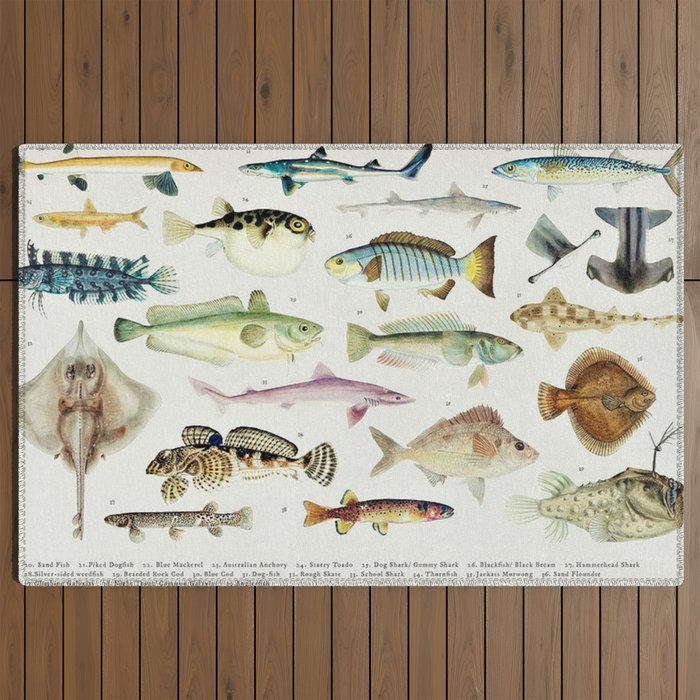The image is a photograph of a poster with a white background, hanging on a finely maintained wooden interior wall. The poster features numerous illustrations of different types of fish—approximately 15 to 20 in total. The illustrations display a variety of fish, including long fish, an eel, a puffer fish, an angler fish shown from the side, a hammerhead shark, a flounder, and other conventional and unusually shaped fish. Some of the fish are depicted from a top-down perspective, and some are just heads of fish, adding to the poster's eclectic look. The illustrations have an old-fashioned aesthetic. Below the fish, you can find a numbered list of names in black text, correlating each fish with its respective name. There is also some additional text or possibly design elements along the sides of the poster, though they are too small to read clearly.